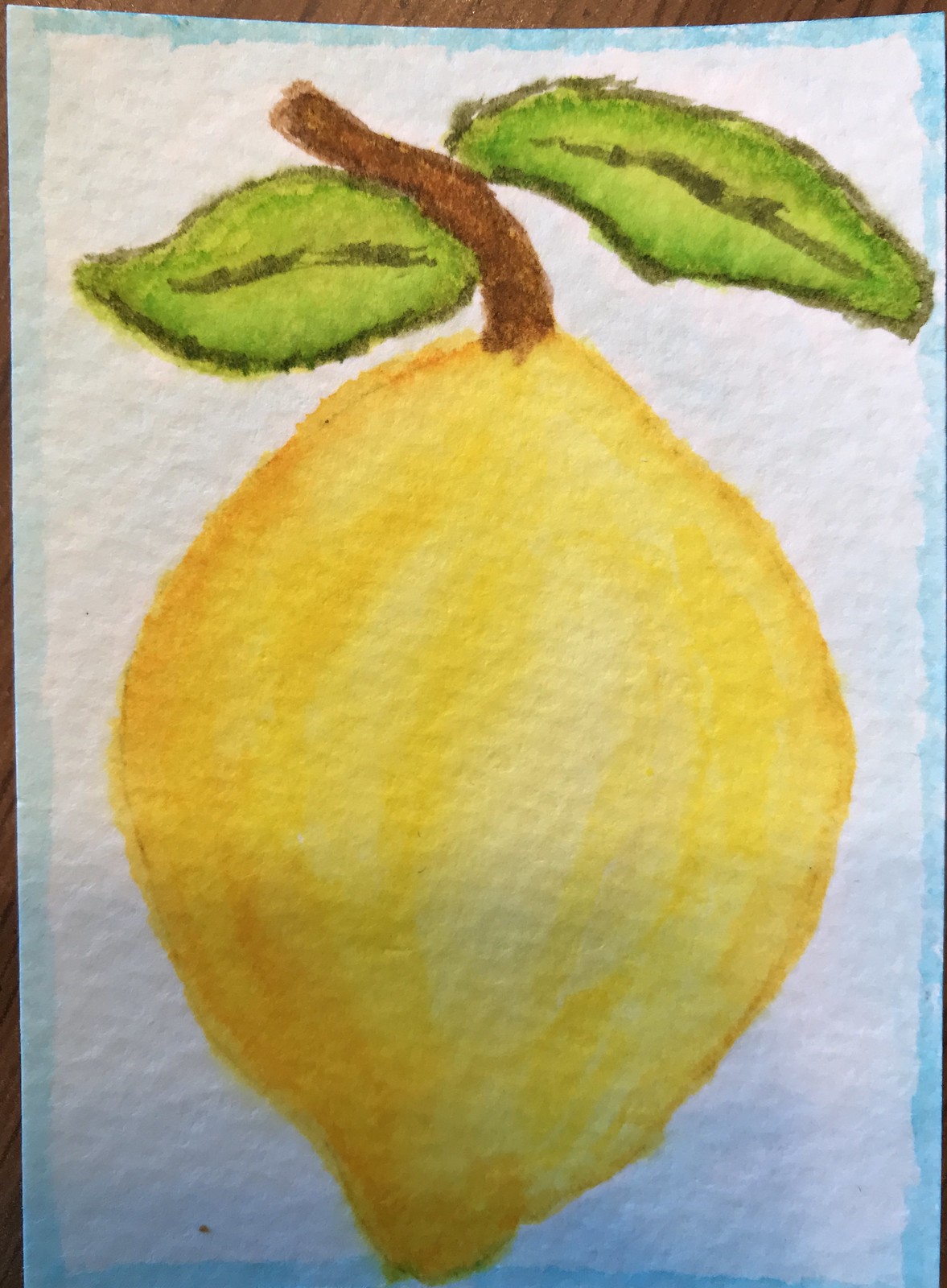This close-up image depicts a meticulously drawn lemon, showcasing its vibrant and diverse shades of yellow, light yellow, and gold. The striking brightness of the lemon is accentuated by a brown stem, from which two distinct green leaves elegantly extend from opposite ends. The backdrop features a predominantly white surface, bordered by a soft blue outline, with a hint of the brown table peeking through beneath. This detailed illustration captures the essence and vivid hues of the lemon, set against a subtly contrasting background.